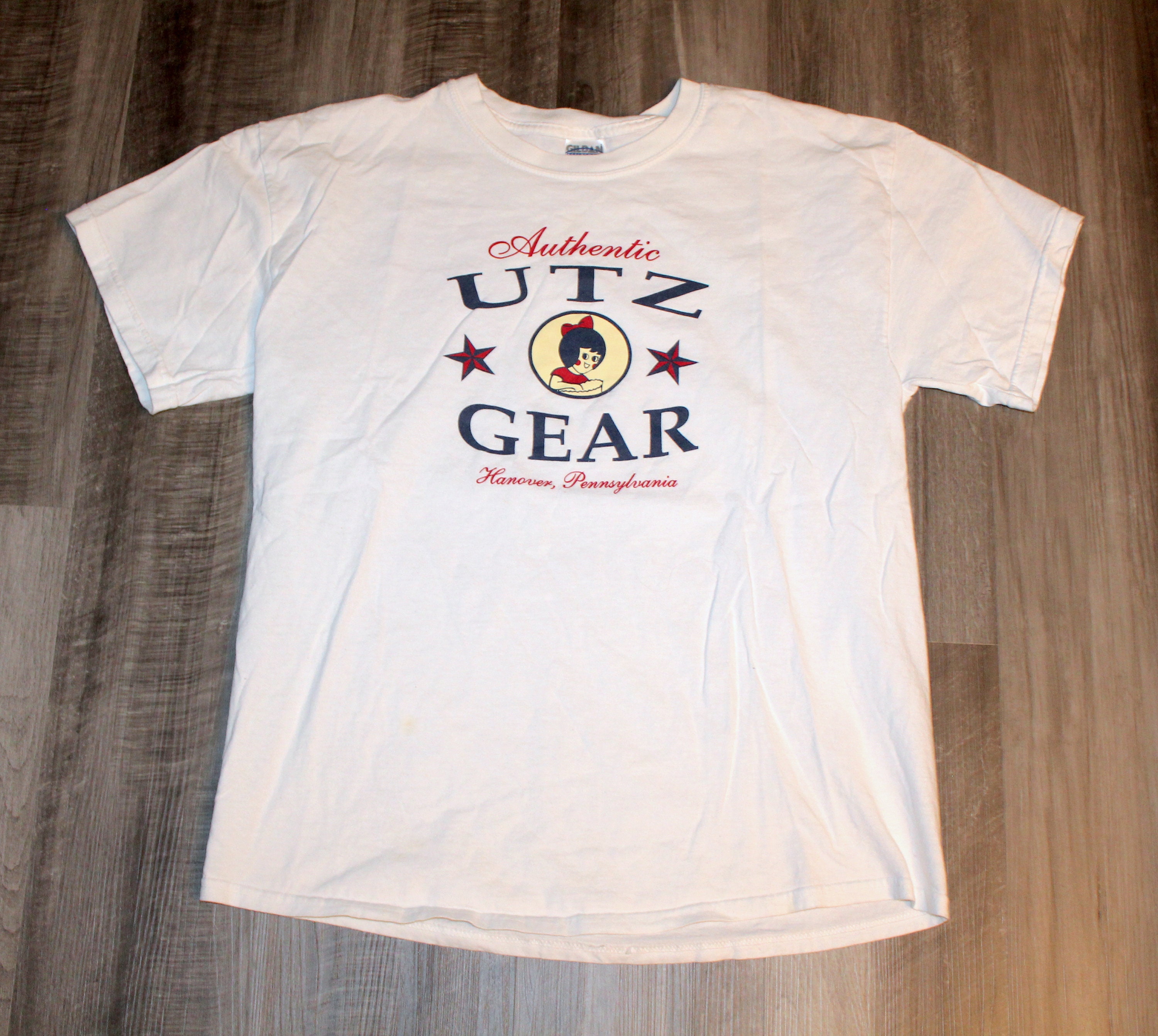This is a square image featuring a white t-shirt laid out on a wooden floor, which appears to be new wood paneling rather than real hardwood. The t-shirt is slightly wrinkled, as if it just came out of a box. In the center of the t-shirt, "Authentic" is written in red script, with "Utz Gear" in blue block letters directly below it. At the bottom, it says "Hanover, Pennsylvania." Separating the words "Utz" and "Gear" are two stars, one red and one blue, flanking a round emblem. The emblem features a cream-colored background with a cartoon character of a little girl with black hair, a red bow, and red cheeks. She is depicted wearing a red shirt and has her hand inside a bag. The tag on the back of the t-shirt indicates it is a Gildan brand. This detailed design suggests the shirt is a commemorative piece celebrating Utz, potentially the snack brand from Hanover, Pennsylvania.